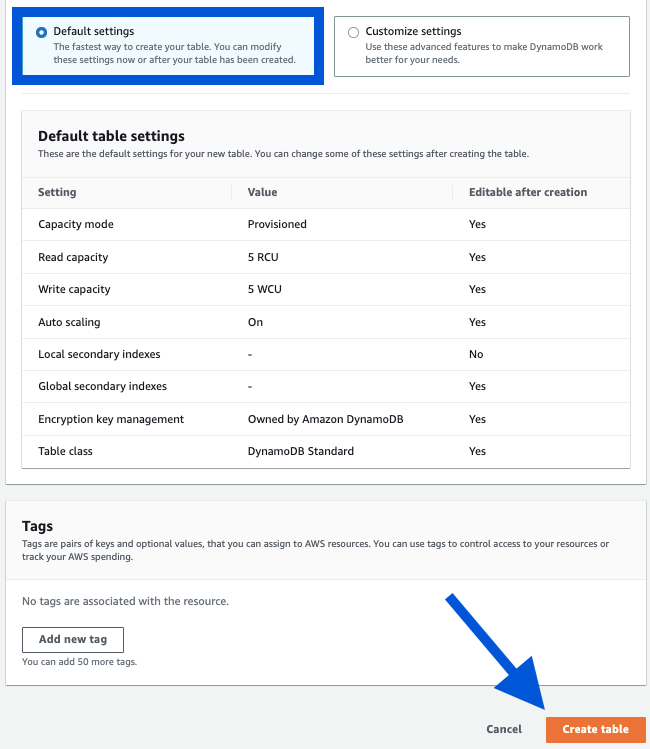The image is a screenshot of a settings page for creating a table in DynamoDB, characterized by its organized layout and detailed options. In the top left corner, encapsulated by a thick blue border, the "Default settings" option is visibly selected with a blue circle indicator. This option highlights that it is the fastest way to create a table and notes that these settings can be modified either now or after the table is created. To the right, the "Customize settings" option remains unselected and suggests using advanced features for enhanced customization of DynamoDB according to specific needs.

Beneath these options, in bold, the text reads "Default table settings," informing the user that these predefined settings can be adjusted post-creation. The page is divided into three columns with headings: "Setting," "Value," and "Editable after creation." 

There are eight specific settings listed below:
1. **Capacity mode:** Set to "Provisioned," and it is editable.
2. **Read capacity:** Set to "5 RCU," and it is editable.
3. **Write capacity:** Set to "5 WCU," and it is editable.
4. **Auto scaling:** Set to "On," and it is editable.
5. **Local secondary indexes:** marked with a dash, indicating it is not editable.
6. **Global secondary indexes:** marked with a dash, indicating it is editable.
7. **Encryption key management:** Managed by "Amazon DynamoDB," and it is editable.
8. **Table class:** Set to "DynamoDB Standard," and it is editable.

A separate section labeled "Tags" explains that tags are pairs of keys and optional values that can be assigned to AWS resources. It also notes that no tags are currently associated with this resource and provides an option to add a new tag.

At the bottom right corner of the page, a prominent blue arrow points directly to the "Create Table" button, suggesting the next step for the user to complete the setup.